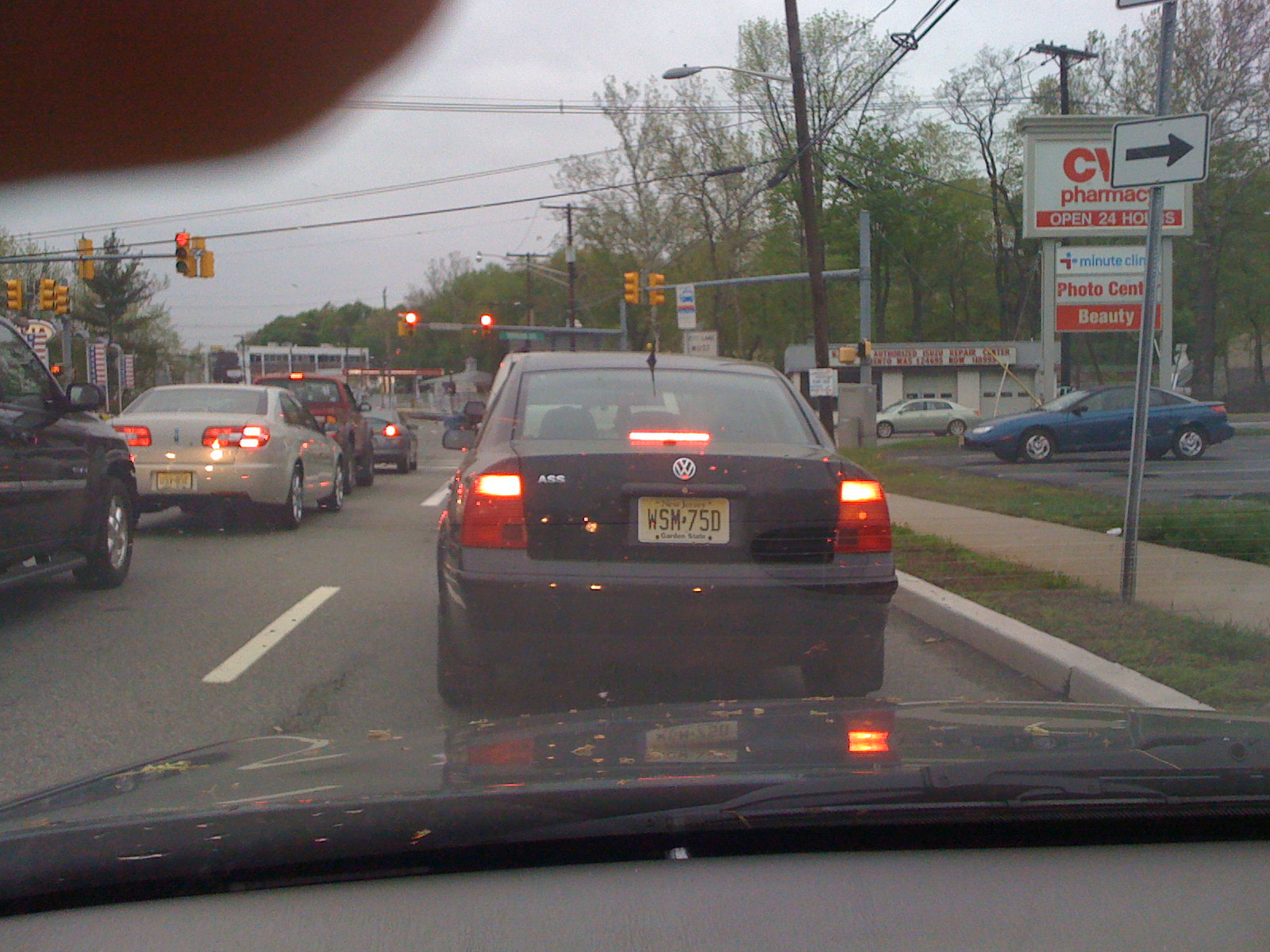Photographed from the inside of a car waiting at a stop sign, this image captures a scene from a two-lane road, presumably taken about a decade ago judging by the signs. The car is positioned four or five vehicles behind the front of the line at a red light. Prominent in the image is a CVS Pharmacy store, distinguished by its signage that reads “CVS Pharmacy, open 24 hours,” and advertises additional services like a MinuteClinic and a photo center. The parking lot of the CVS is bustling, with an older model Camaro notably parked out front. Across from the CVS, a garage can be seen, emphasizing the rural nature of the area, which is further highlighted by a line of trees in the background. Directly in front of the photographer's car is a black Volkswagen, bearing a yellow and black license plate that appears blurred, making it difficult to determine the issuing state.